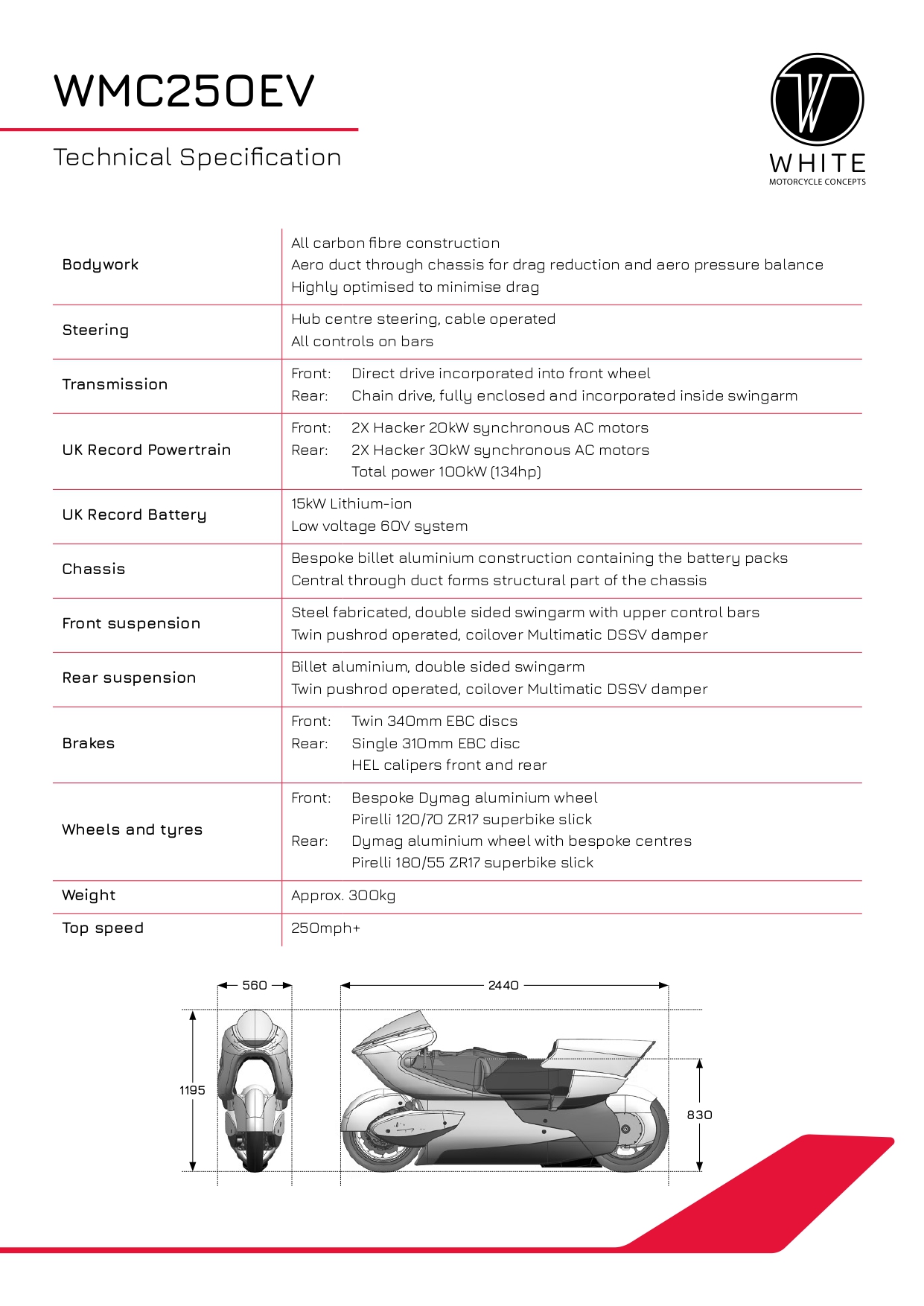The image depicts a detailed technical specifications page for the WMC250EV motorcycle model. Set against a white background, the top features the bold, underlined title "WMC250EV technical specifications." In the top right corner, a black circular logo with a stylized "W" and the text "White Motorcycle Concepts" is present. The layout is organized into two columns: the left column lists various features such as bodywork, steering, transmission, UK record powertrain, UK record battery, chassis, front and rear suspension, brakes, wheels and tires, weight, and top speed. The right column provides detailed descriptions of these features. Notably, the bodywork includes all carbon fiber construction with an aero duct through the chassis for drag reduction and aero pressure balance, and the steering utilizes hub center steering with cable-operated controls on the bars. The bike boasts a top speed of over 250 miles per hour. At the bottom of the page, there are illustrations of the motorcycle in both profile and head-on views, showcasing its sleek design with an elongated seat, tail wing, and distinctive aero features. The bike's color scheme is predominantly gray and black, complemented by a black seat. The document is densely packed with technical data, emphasizing the high-performance engineering of the WMC250EV.